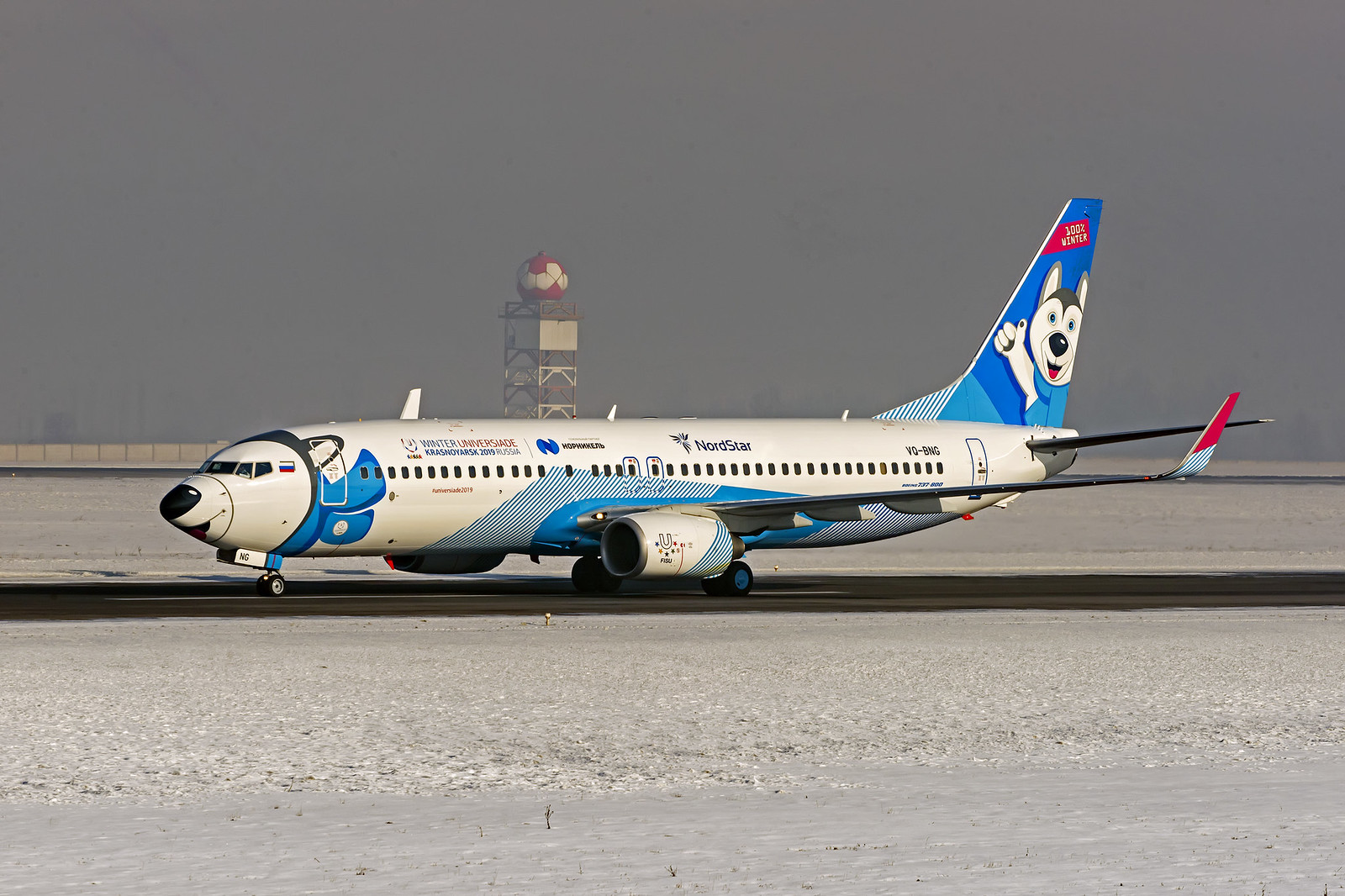An airplane is parked on a snow-covered runway, the only clear area amidst a cold, wintry landscape. The front of the plane is creatively painted to resemble a husky mascot, complete with a cheerful, cartoonish appearance. The husky, depicted with blue eyes and wearing a scarf, is shown giving a thumbs-up from the top fin of the plane. The aircraft’s nose is painted black to mimic the husky's snout, with a painted mouth underneath. The cockpit windows are integrated into the design, representing the husky's eyes. The background is overcast with thick, gray clouds, emphasizing the cold atmosphere. A control tower looms in the distance, partially visible through the cloudy haze.